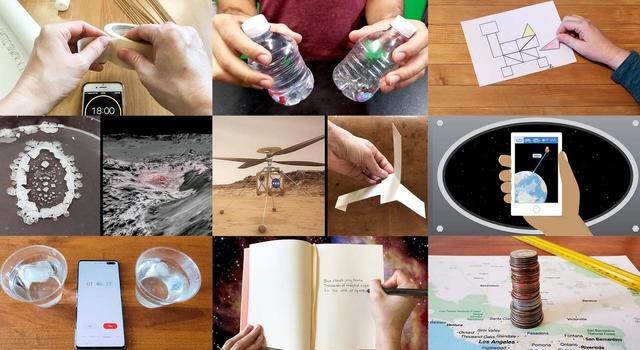This image collage consists of 11 distinct, detailed images arranged in a grid pattern. The top row features three larger rectangular images. Starting from the left, the first shows a person with pale skin, tearing off a piece of masking tape while a phone displaying "18 minutes" rests on the table below. The middle image captures a man in a burgundy shirt, holding two small water bottles, one in each hand. The last image in the top row depicts a hand placing colorful shapes, including a pink triangle, onto a piece of paper laid on a wooden surface. 

The second row contains five varied images. On the far left, a circular beach scene with sand or shells is shown, followed by an adjacent image resembling craters on the moon, with some pink hues. Next, there is a depiction of a drone-like aircraft with propellers, situated in a desert-like terrain. Continuing, another image shows hands manipulating a paper origami crane on a wooden background. The final image in this row is an animated depiction of a person holding a tablet displaying an Earth map with a satellite, set against a black oval backdrop.

The bottom row comprises three images. The first depicts a phone with a timer on a wooden table, flanked by two water glasses possibly containing ice. The middle image showcases a book open on a starry backdrop, with someone writing in it using their right hand and a black pen. The last image presents a map on a brown table, adorned with a stack of coins and a yellow ruler, creating a scene suggestive of navigation or planning.